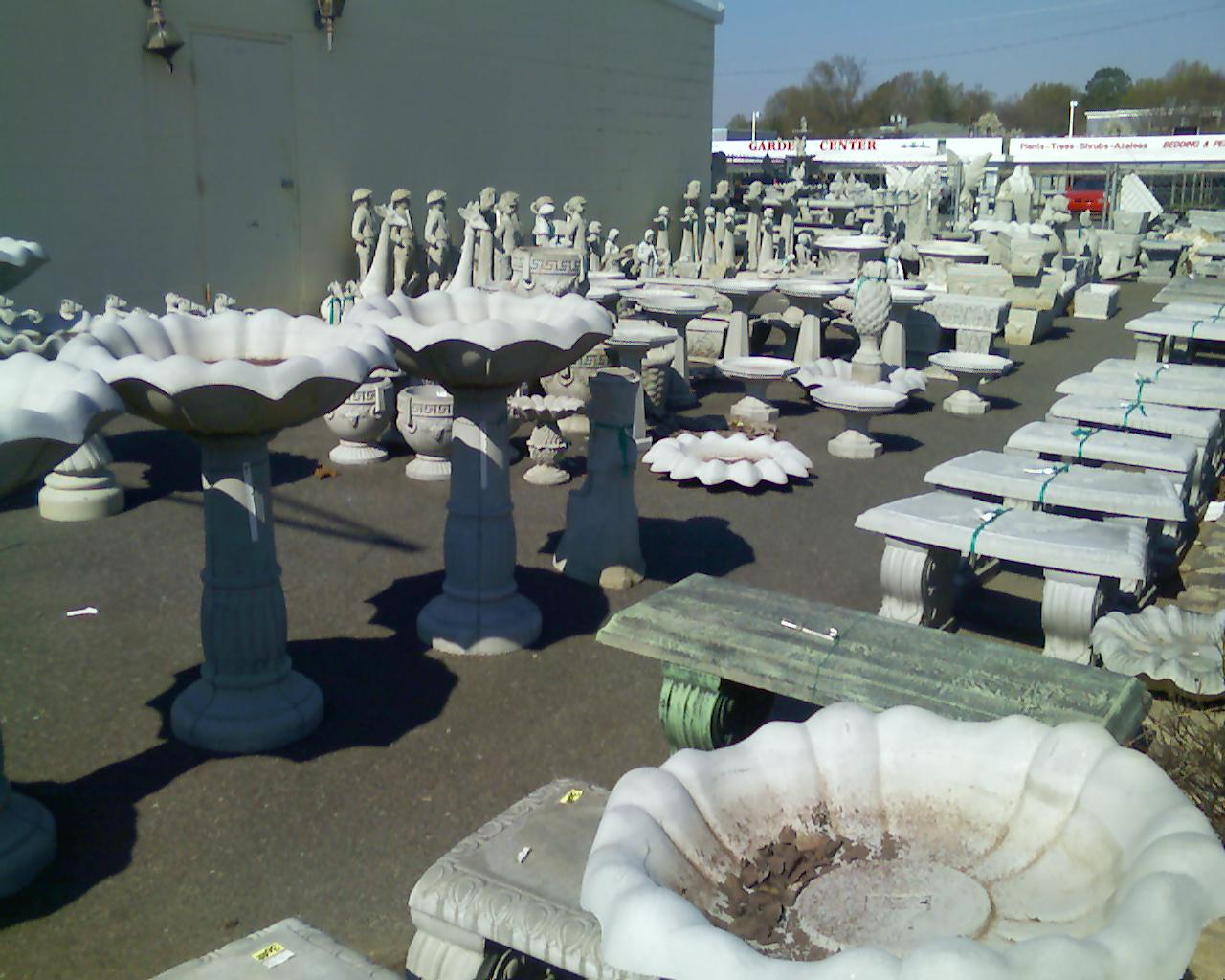This photograph captures a large outdoor lot brimming with an extensive array of stoneworks and garden decorations. The space is teeming with numerous items carved from gray granite-like stone, including water fountains, large birdbaths, and various statues—some of which are sculpted into elegant human figures. Rows of meticulously crafted stone benches stretch across the lot, interspersed with ornate columns, chalice-shaped stone bowls, and pots. Each piece seems designed to enhance garden aesthetics or serve functional purposes in outdoor spaces. Towards the back, a white banner with bold red text identifies a "Garden Center," suggesting a nearby road with additional shops, highlighting the area's focus on garden utilities and decorations. The scene is set under a slightly overcast sky, perhaps indicating an approaching dusk, which casts a muted light over the stone inventory, enhancing the tranquil and timeless atmosphere.